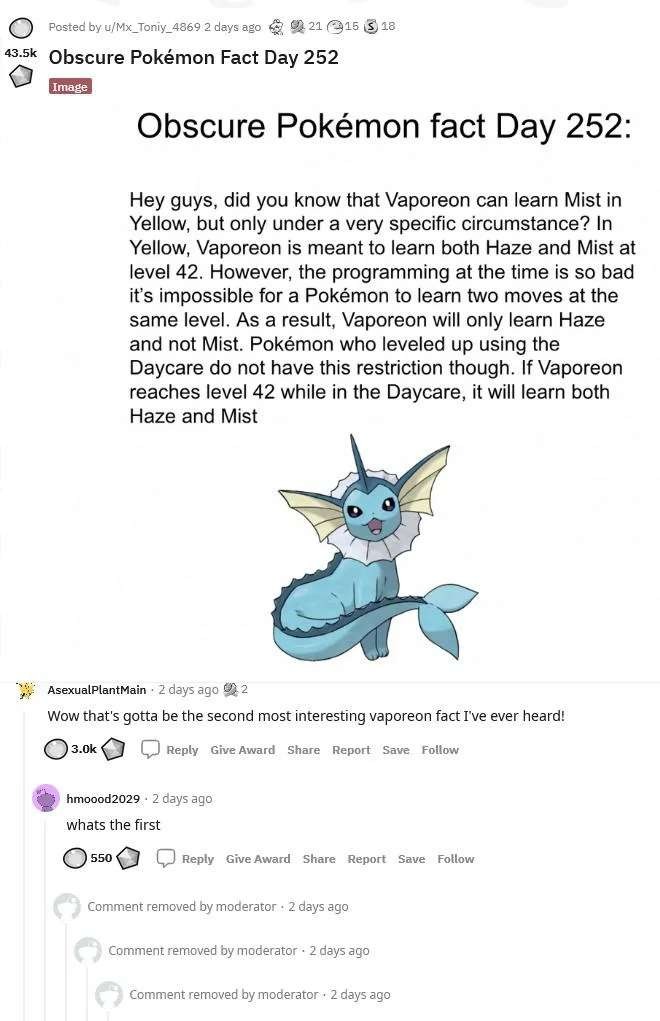**Image Description:**

A vertical rectangle image, seemingly a social media post, potentially sourced from a platform like Reddit. 

- **Header:** At the very top left corner, the text reads, "Posted by u/mxtonemy 2 days ago". Alongside this, various social media icons are scattered.
- **Main Content:** Below the header, there's a bold title stating, "Obscure Pokémon Fact Day 252." This title is repeated below, emphasizing the subject.
- **Body Text:** The detailed content provides an interesting Pokémon fact about Vaporeon:
  
  "Hey guys, did you know that Vaporeon can learn Mist in Yellow, but only under a very specific circumstance? In Yellow, Vaporeon is meant to learn both Haze and Mist at level 42. However, due to programming limitations at the time, it's impossible for a Pokémon to learn two moves at the same level. As a result, Vaporeon will only learn Haze and not Mist. Pokémon leveled up using the Daycare do not have this restriction, though. If Vaporeon reaches level 42 while in the Daycare, it will learn both Haze and Mist."
  
- **Visuals:** Accompanying the text, there is an image of Vaporeon. The creature is depicted with cat-like features, large ears, a fin protruding from its head, and a distinctive fish or whale-like tail.
  
- **Comments:** Below the informational content, there are comments from users. One noteworthy comment reads, "Wow, that's got to be the second most interesting Vaporeon fact I've ever heard."

This detailed caption provides a comprehensive understanding of the post's content and its visual elements.